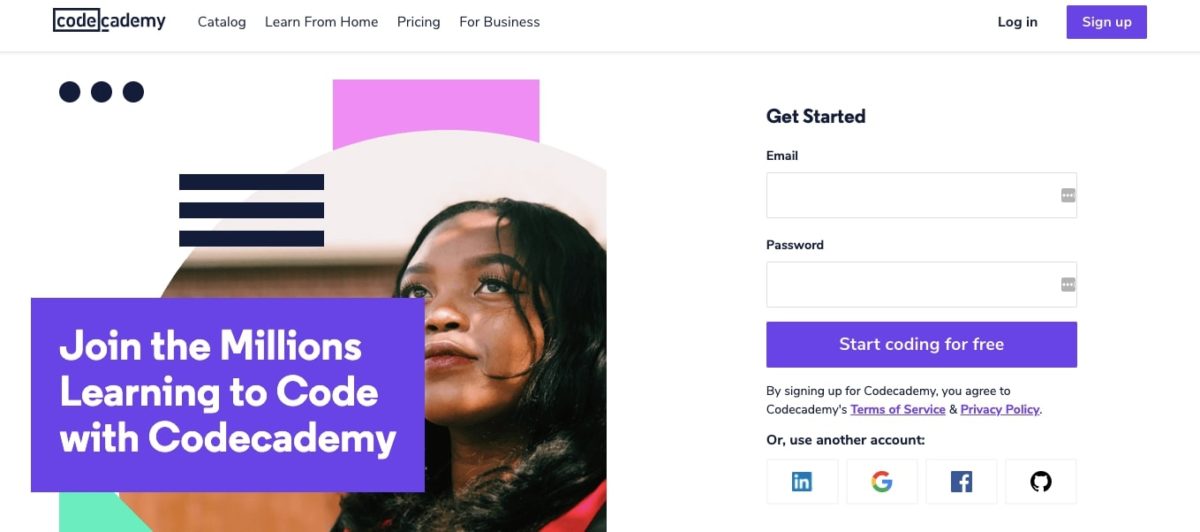The homepage of Codecademy features a clean, minimalist design with a predominantly white background and black text. At the top of the page, there are several links: "Catalog," "Learn From Home," and "Pricing for Business." On the right side of the navigation bar, users can find options to "Log In" or "Sign Up," with the "Sign Up" button highlighted in a purplish color.

The Codecademy logo is simple yet distinctive, featuring the word "Codecademy" with "code" enclosed in a box. Below the navigation bar, a stock photo of a young Black woman gazing into the distance is prominently displayed. Overlaying the image is text that reads, "Join the millions learning to code with Codecademy."

To the right of the image, there is a form where users can get started by entering their email and creating a password. A purple button labeled "Start Coding For Free" is provided to initiate the sign-up process. Additionally, users have the option to log in using accounts from LinkedIn, Google, Facebook, or GitHub. Links to the Terms of Service and Privacy Policy are also available.

Codecademy offers tutorials and classes in various programming languages, designed to facilitate coding education. The site's user interface is minimal and free of clutter, ensuring an efficient and straightforward user experience.